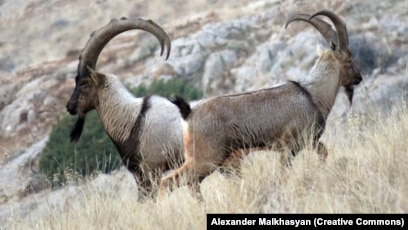This image features two majestic Bezoar goats with long, curved horns that arc back gracefully. Both goats exhibit distinctive coloring: the one in the foreground, looking to the right, has predominantly whitish-gray fur with a dark face and a striking black stripe across its shoulder, while the one in the background, looking to the left, has similar markings but with a darker, grayish-brown body and a lighter beige neck. They are standing on a grassy, rocky hillside, surrounded by tall, beige grass and a mix of green and brown bushes and shrubs in the background. The foreground goat's antlers are slightly more pronounced. The image is a Creative Commons work by Alexander Malkhasyan.